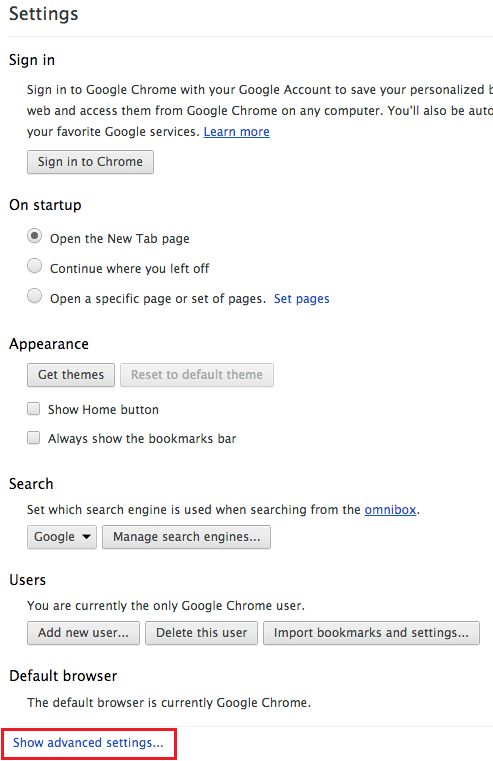The image displays a settings page for Google Chrome, guiding users on various customization options and sign-in processes. At the top, there is a prompt to sign into Google Chrome using a Google account, enabling password saving, web access synchronization across devices, and automatic usage of favorite Google services. The prompt includes a "Learn more" link and a "Sign into Chrome" button.

In the "On Startup" section, users can choose between three options: open the New Tab page, continue where they left off, or open a specific set of pages. The pages currently set to open are designated as the New Tab page.

The "Appearance" section features options to get new themes or reset to the default theme. There are also toggle settings for showing the home button and always displaying the bookmarks bar.

The "Search" section allows users to set their preferred search engine to be used from the Omnibox, with Google as the default. There is a dropdown menu to choose other search engines and a "Manage search engines" button, both enclosed in grey boxes.

Under "Users," it indicates that the current user is the only one using Google Chrome. Options available include adding a new user, deleting the current user, and importing bookmarks and settings.

Finally, the "Default Browser" section confirms that Google Chrome is currently the default browser. There is also an option to "Show advanced settings" for further customization.